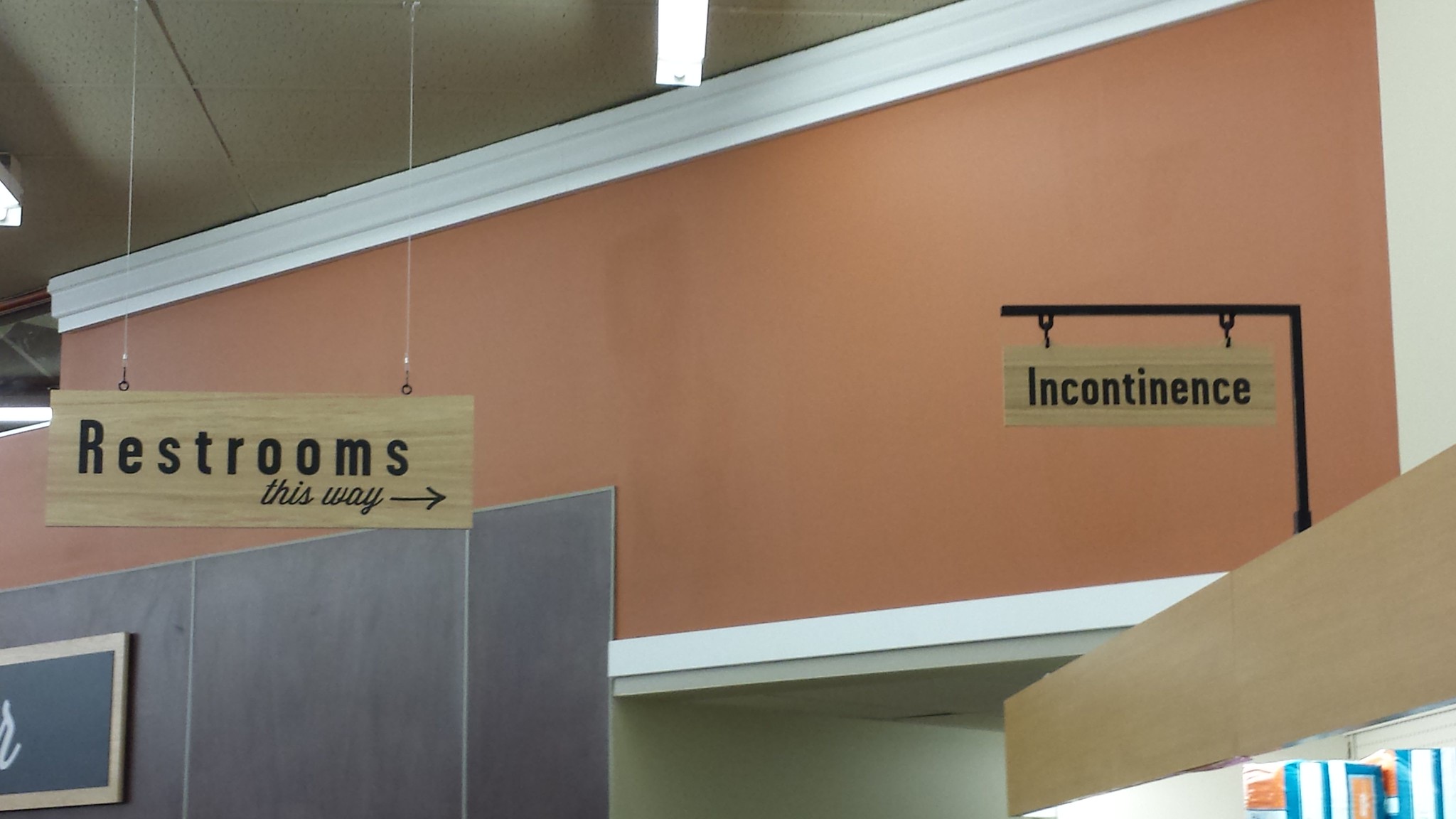This is a detailed color photograph of the interior of a commercial establishment, captured in landscape mode. The room features white crown molding along the ceiling and rust-colored walls, with an additional blue wall visible behind some signage. Hanging from the ceiling on thin white ropes is a light-colored wooden sign with black lettering that reads "Restrooms this way" accompanied by an arrow pointing to the right, directing towards a partially visible doorway. To the right of this sign, there's an oblong wooden sign suspended from a black, upside-down L-shaped frame with the word "Incontinence" in black letters, indicating an area likely related to personal hygiene products. At the bottom right corner of the image, a beige structure is seen alongside a blue and white element that might be part of a shelf or display. The entire scene is lit by fluorescent lights, and the presence of these two prominent signs helps define the surrounding space as a room in a retail store, though the exact nature of the store remains unspecified. The photograph meticulously avoids including any people, animals, vehicles, plants, or floral elements.